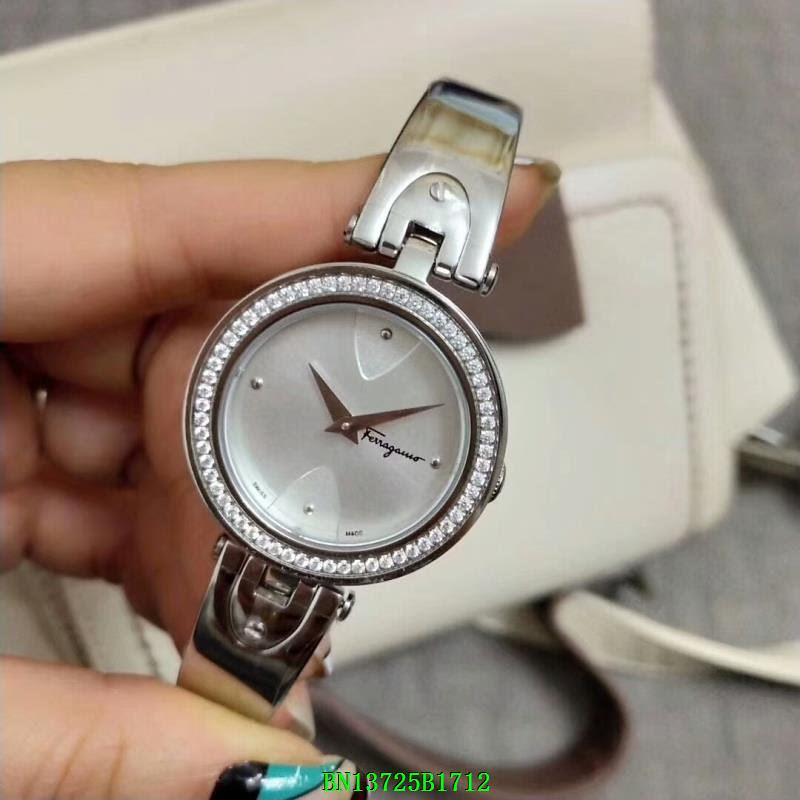This image features a luxurious Ferragamo watch, characterized by its opulent design. The watch boasts a striking silvery-white face adorned with a precise row of tiny, shimmering diamonds encircling it. Complementing its elegant appearance, the timepiece has a sophisticated silver band. The watch face is uncluttered, marked only by silver dots at the 12, 3, 6, and 9 o'clock positions, providing a minimalist, yet refined aesthetic. The black, pointed hands indicate the time as either 10:10 or 11:10, adding to the watch's timeless elegance. On the right side, a small knob can be seen. The watch is being gently held by someone’s left hand, highlighting its size and adding a personal touch to the image.